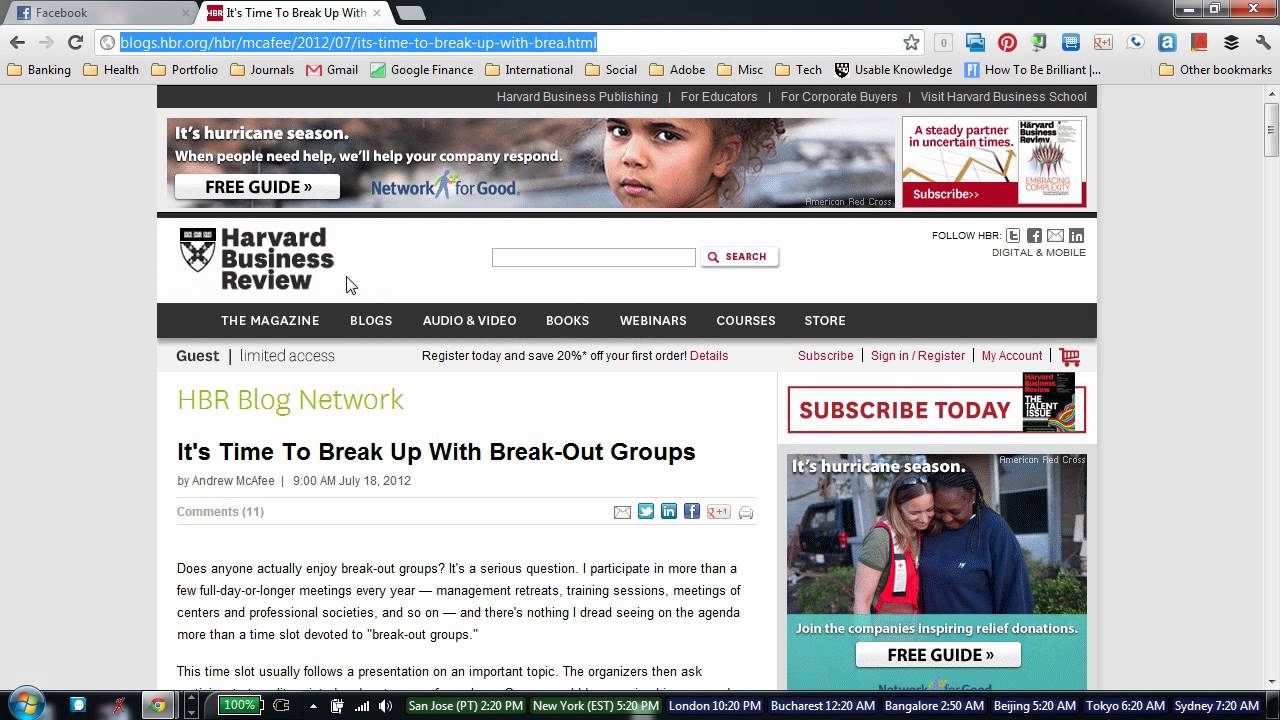This screenshot captures a desktop browser with two open tabs. The tab on the left displays Facebook, while the tab on the right displays a blog from the Harvard Business Review (HBR). The blog is titled "It's Time to Break Up with Breakout Groups." 

The browser's address bar shows the URL of the HBR article, highlighted in blue, indicating that it has been selected. At the top of the HBR web page, there's a horizontally aligned advertisement stating, "It's hurricane season - Free guide from the Network for Good."

Directly beneath the advertisement is the HBR header, which includes the HBR logo located at the top left. Centrally positioned is a search bar, followed by a black banner showcasing various categories: The Magazine, Blogs, Audio and Video, Books, Webinars, Courses, and Store. 

Below this banner is a green-highlighted label indicating the "HBR Blog Network." The article's title, "It's Time to Break Up with Breakout Groups," is prominently displayed in bold black print. The content of the article appears just below the title.